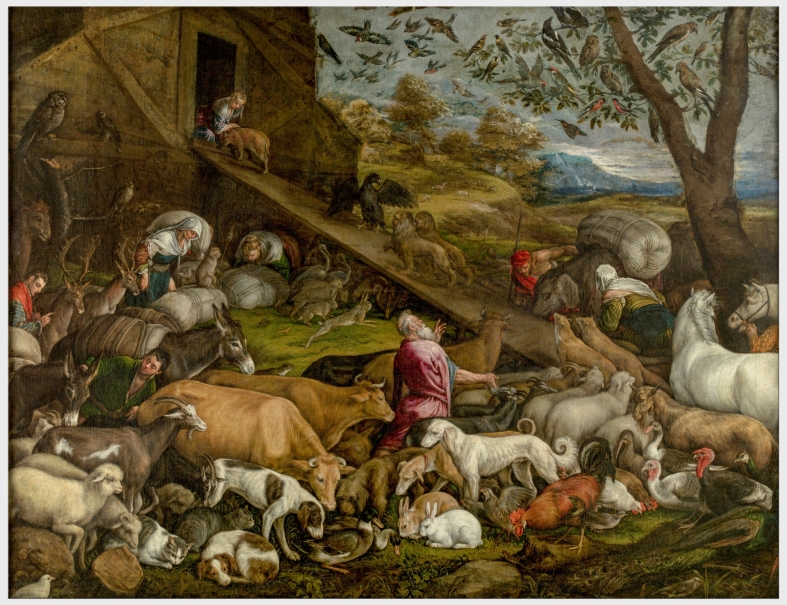The painting is a detailed biblical depiction of Noah's Ark, with a landscape that is broader than it is tall. At the center-bottom, Noah is prominently featured, an elderly man with gray hair and beard, wearing a long red robe. His hands are raised, and his head tilts skyward as if he is proclaiming something. Surrounding Noah are numerous animals being ushered by several people scattered throughout the scene. The animals, a diverse assembly including cows, dogs, sheep, horses, donkeys, rabbits, chickens, and roosters, are positioned in layers, almost stacked upon each other. 

A ramp begins approximately a third up the image on the right-hand side, sloping diagonally towards the upper left corner, leading to the second story of a large brown barn, which serves as the ark. The sky above is painted in dark gray and bluish hues, indicating an impending storm, and is populated with numerous birds in flight, adding to the sense of urgency and chaos. There's also a tree beneath the flying birds, adding to the biblical atmosphere. The image captures the essence of the moment as people and animals prepare for the deluge, emphasizing the meticulous and frenetic preparation for the coming flood.